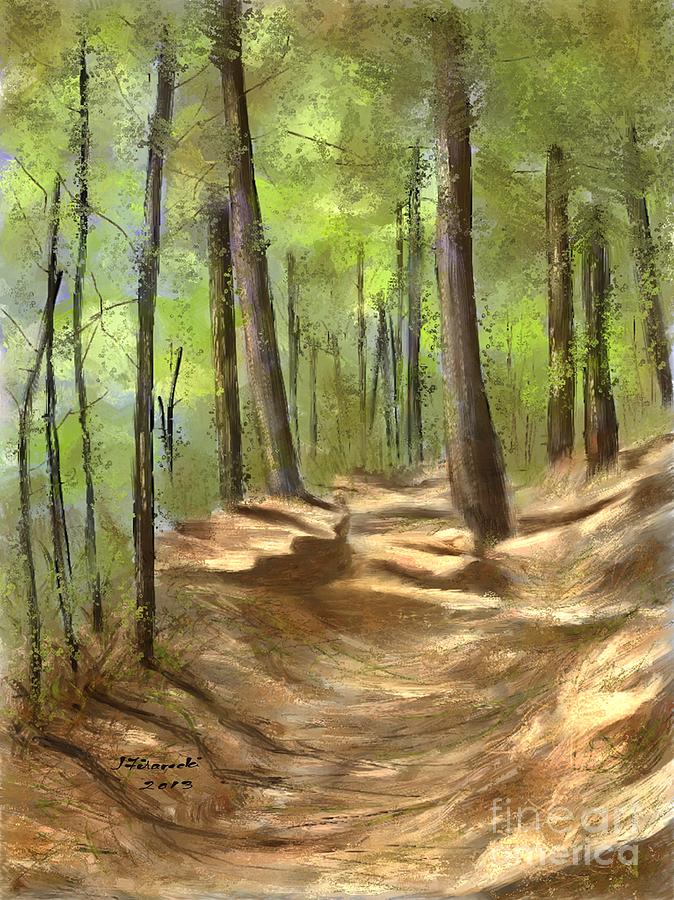This painting depicts a serene forest scene, characterized by a dusty, winding trail that progresses upwards through the wooded area. The style of the painting has an almost impressionist influence, with delicate brushwork and visible textured lines that suggest an artist's hand actively working the medium. The trail itself is a mix of brown and beige tones, bordered by tall trees with bark ranging from dark brown to light grey. The light green leaves add a vibrant contrast, their hues shifting from a lime shade to a deeper forest green, occasionally tinged with brown at the tips. The forest floor consists of a rough, dirt-like terrain, with shadows cast by the trees indicating an afternoon setting. Prominently, there are major trees flanking the trail with thinner trees on the left and wider trees in the background. This horizontal landscape format captures the natural beauty of the forest, highlighting both the depth and texture of the woodland environment. Additionally, the painting contains a signature on the left side and a "Fine Art America" watermark in the lower right corner, subtly marking its artistic provenance.